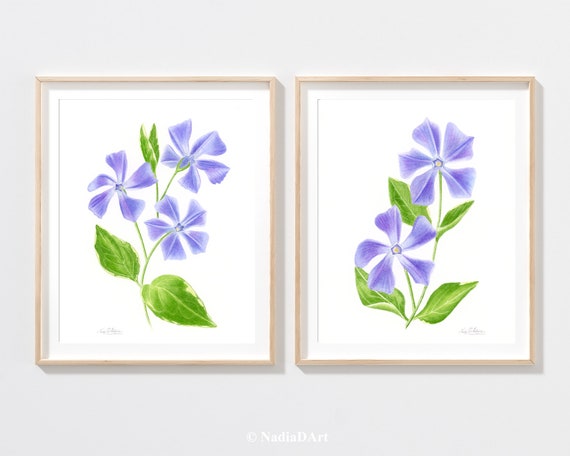This image features two rectangular paintings, slightly taller than they are wide, hung side by side on a white wall, each encased in thin, light wood frames with white matting. The paintings depict purple flowers with green stems and leaves, sharing a similar artistic style but with slight variations. The left painting showcases three light purple flowers with white centers, each with five delicate petals marked by a crease down the middle. These flowers stem from a single branch, accompanied by two leaves at the bottom and one smaller leaf positioned in between the flowers. The right painting, slightly less intricate, displays two similar flowers with four associated leaves—two situated at the bottom and another pair between the blooms. Both pieces are signed "Natya D. Arch," accompanied by a copyright symbol at the bottom. The consistent floral motifs and harmonious presentation create a cohesive and serene visual experience.